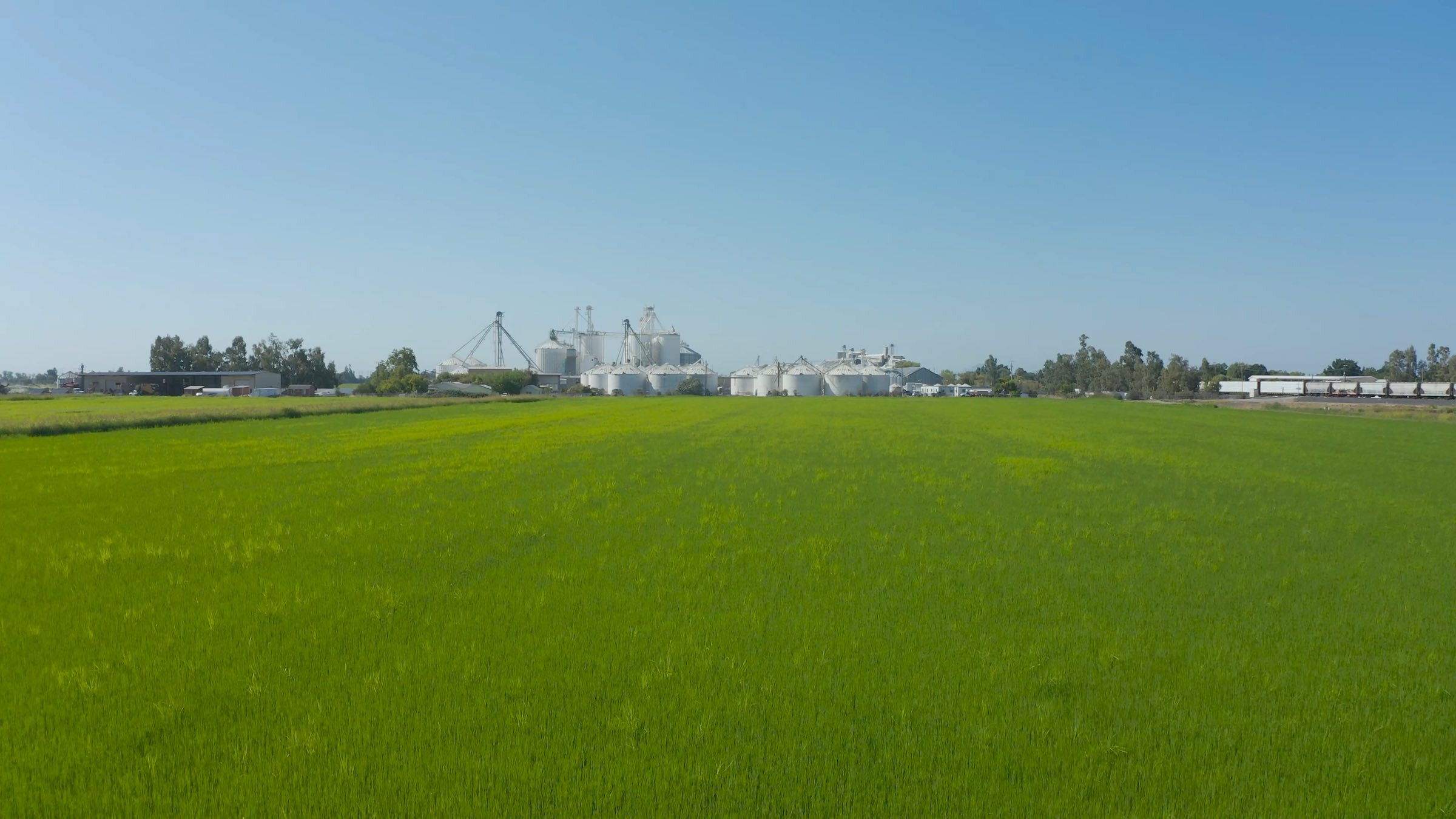This image is a realistic, horizontally oriented photograph showcasing a vast, flat, and vibrant green field under a clear, sunny, blue sky. The grass extends uniformly across the frame, and the horizon line divides the image roughly in the middle. In the background, a series of white silos with round bases and conical roofs are evident, typically used for grain storage on farms. Adjacent to these silos are long, low buildings, likely for farm equipment, storage, or livestock, with the absence of windows suggesting their functional design. Some structures resemble metal scaffolding or conveyor belts leading up to the silos, indicating industrial activity related to an agricultural farm. Additionally, there is a train line visible on the far right, suggesting connectivity for distributing farm products. Trees line the horizon, adding a rural charm to the scene, with no signs of urban development, capturing the serene and open expanse of a farming area.